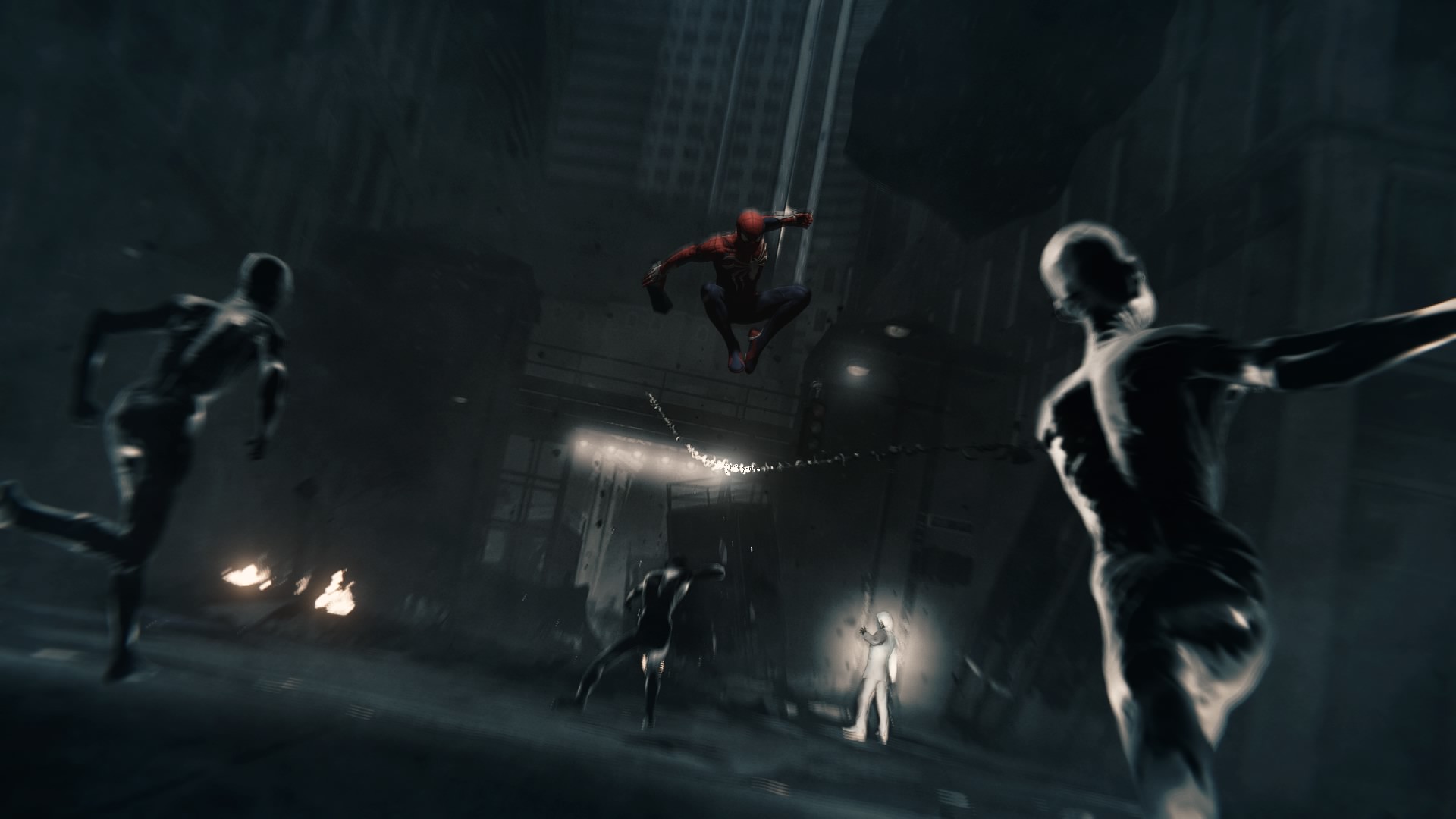In this detailed still from a video game, Spider-Man is captured mid-jump at the center of the screen, illuminated dramatically from above which makes his iconic red and blue suit stand out. He is descending with bent knees and arms outstretched, poised for an imminent attack. Below him, a group of enemies is running towards him, their backs visible to the viewer. These enemies are humanoid mutants, bald and unsettling, with one particularly noticeable figure dressed in glowing white at the immediate center of the action. This white-clad figure appears to be slightly stretching its arm, possibly in defense against Spider-Man’s incoming strike. The scene is urban, with indistinct skyscrapers looming in the background and fires burning on the ground, adding to the chaotic atmosphere. The overall palette of the image is dark and muted, dominated by shades of black and gray, with Spider-Man's vibrant costume providing the only splash of color.